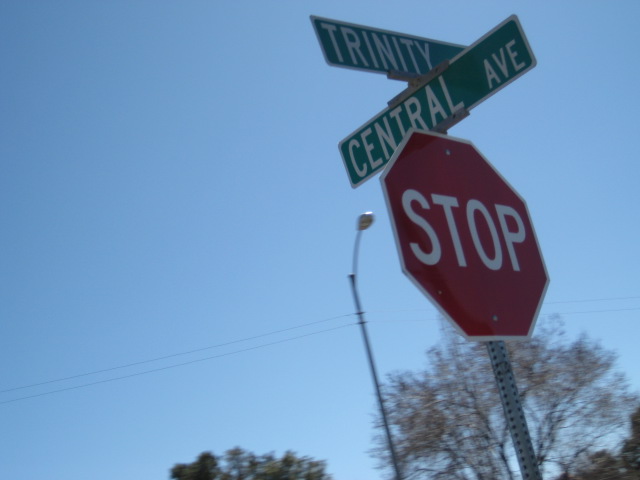This vibrant daytime image captures a red stop sign fixed to a long, silver metal pole, positioned slightly to the right but dominating the frame from top to bottom. Above the stop sign, two green street signs with white text are visible; the top one says "Trinity," but the second part of the name is partially obscured by the position of the "Central Ave" sign below it. Behind these signs, the sky is a clear, gradient blue, darker at the top and becoming lighter and brighter towards the bottom. The scene includes a tall street light with wires extending diagonally across the image, adding a sense of urban infrastructure. Flanking the stop sign, tall trees stretch upwards—on the left, a green-leaved tree, while to the right, another tree showcases autumnal hues, possibly orange leaves, and further right, a tree with bare branches. The overall upward angle of the photograph allows the viewer to look up into the crisp, cloudless sky, underscoring the beauty of the bright, clear day.